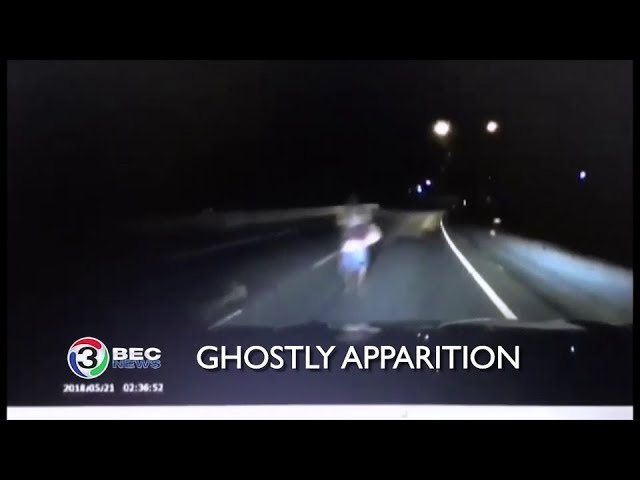The image appears to be a screenshot or photo of a TV screen, displaying a news broadcast from BEC News. The picture shows a dark highway at night, seen from what seems to be the hood or dashboard of a car. The highway's center lines and edges are partially visible, illuminated by the car's headlights. In the middle of the road, there's a very blurry and indistinct figure, which is possibly a person, and is the focus of the broadcast claiming to show a "ghostly apparition." The text "GHOSTLY APPARITION" is prominently displayed in all capital white letters with a black drop shadow, situated above a white banner at the bottom of the screen. On the left side, there's a BEC News logo featuring a black number 3 encircled by red, green, and blue arches. The date and time are also shown but are difficult to discern due to the image's blurriness. The entire broadcast image is bordered by thick black rectangular bars at the top and bottom.